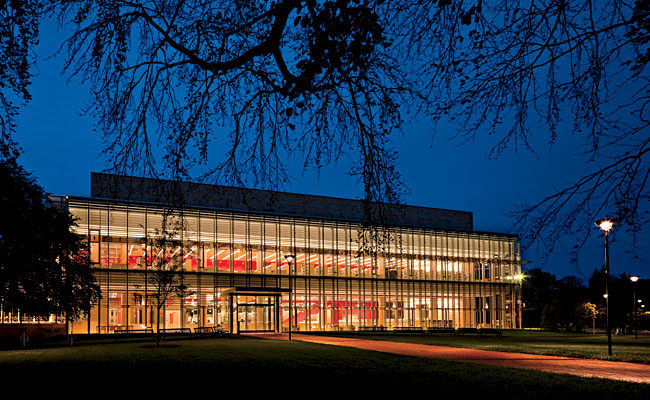The photograph captures the Cambridge Municipal Library, a modern two-story building primarily composed of glass windows, emphasizing its contemporary architectural style. Taken at night, the sky is a deep, dark blue, indicating it is shortly after sunset. The well-lit interior of the library radiates through its clear glass facade, revealing overwrought fluorescent lighting and hints of red signage. The library, nestled in a verdant park-like setting, is approached by a red or maroon brick pedestrian pathway. Street lamps subtly illuminate the area around the building, while overhanging tree branches and bushes frame the scene, casting gentle shadows and adding a natural contrast to the sleek, illuminated structure.